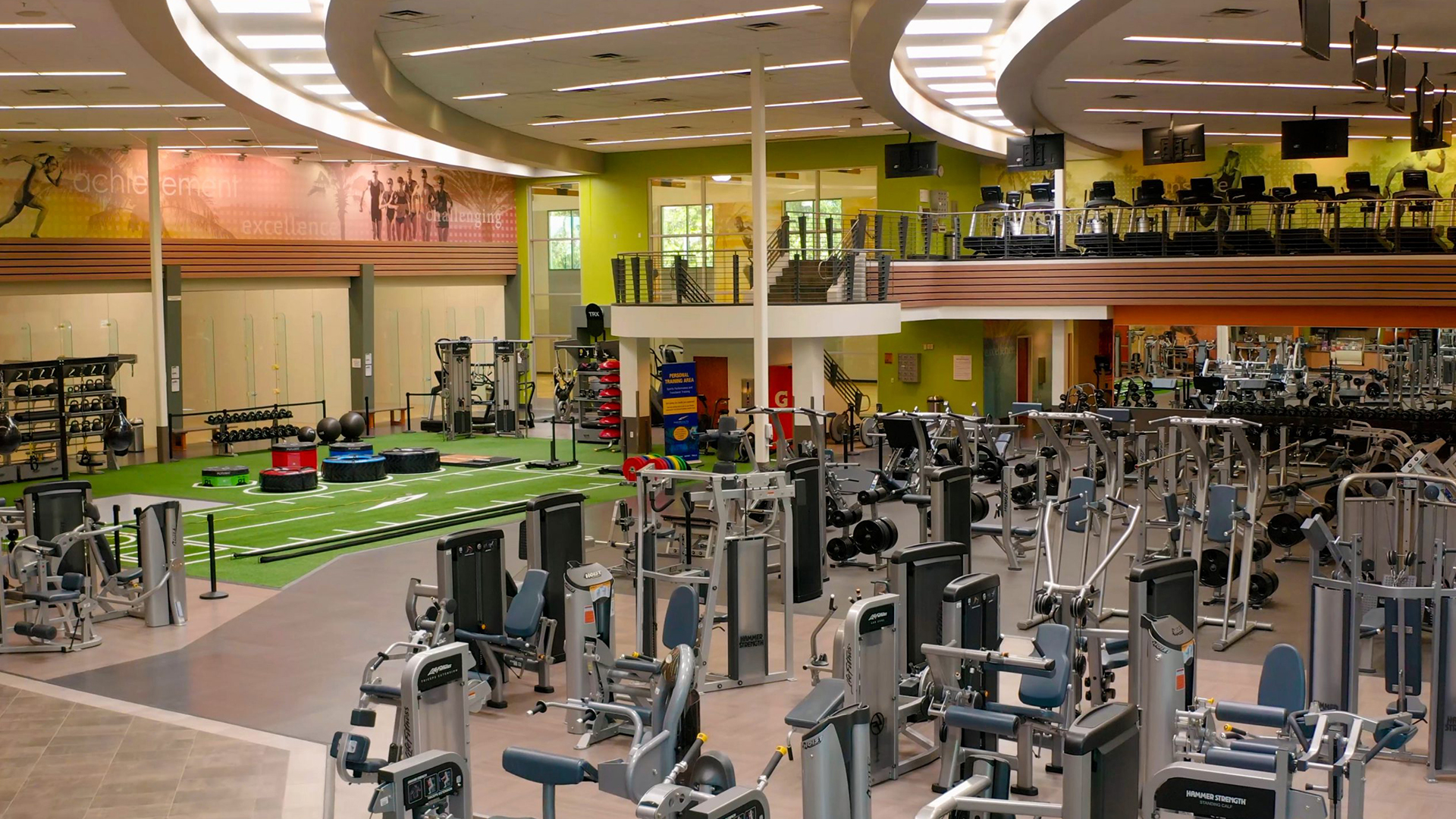This is a detailed color photograph taken inside a spacious, multi-level fitness gym. The image, captured from an elevated vantage point, showcases an extensive array of workout equipment. In the foreground, numerous silver weight machines and exercise equipment are neatly arranged. Toward the left, there is a green mat area designated for weightlifting, complete with a shelf storing various weights and additional weight machines.

The background reveals a set of stairs leading to the second floor, which is dedicated to cardio exercises. This upper level features a wall lined with treadmills, each equipped with televisions hanging from the ceiling. The gym boasts a vibrant and inviting atmosphere, with walls adorned in shades of green, pink, yellow, cream, and chartreuse. Complementing the colorful walls, a mural depicting people running adds an energetic flair to the space. The ceiling is fitted with fluorescent lights, ensuring the area is well-lit. Notably, the photograph captures an empty gym, devoid of people, highlighting the expansive and pristine nature of the facility.